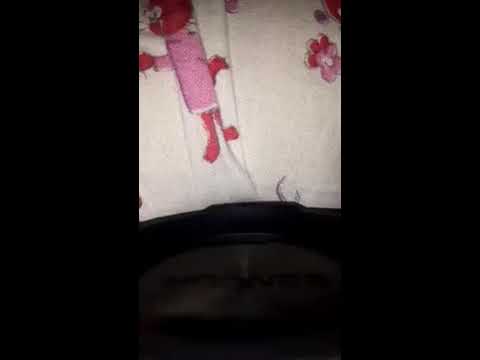This image showcases a white baby blanket adorned with cartoon-like figures, primarily in pink and red. The blanket occupies the center of the photograph, surrounded by thick black bars on the left and right sides, creating a narrow frame. The top of the blanket seems to extend out of the photo's frame, and the foreground features a mysterious black, curved object with indistinguishable lettering. The design on the blanket includes whimsical characters such as a probable animated mouse in a pink dress and other indeterminate animals, possibly including a cat and a dinosaur. The blanket is crumpled and wrinkled, obscuring parts of these illustrations, and a pink flower is partly visible in the pattern. The background and floor are indiscernible, immersed in darkness.